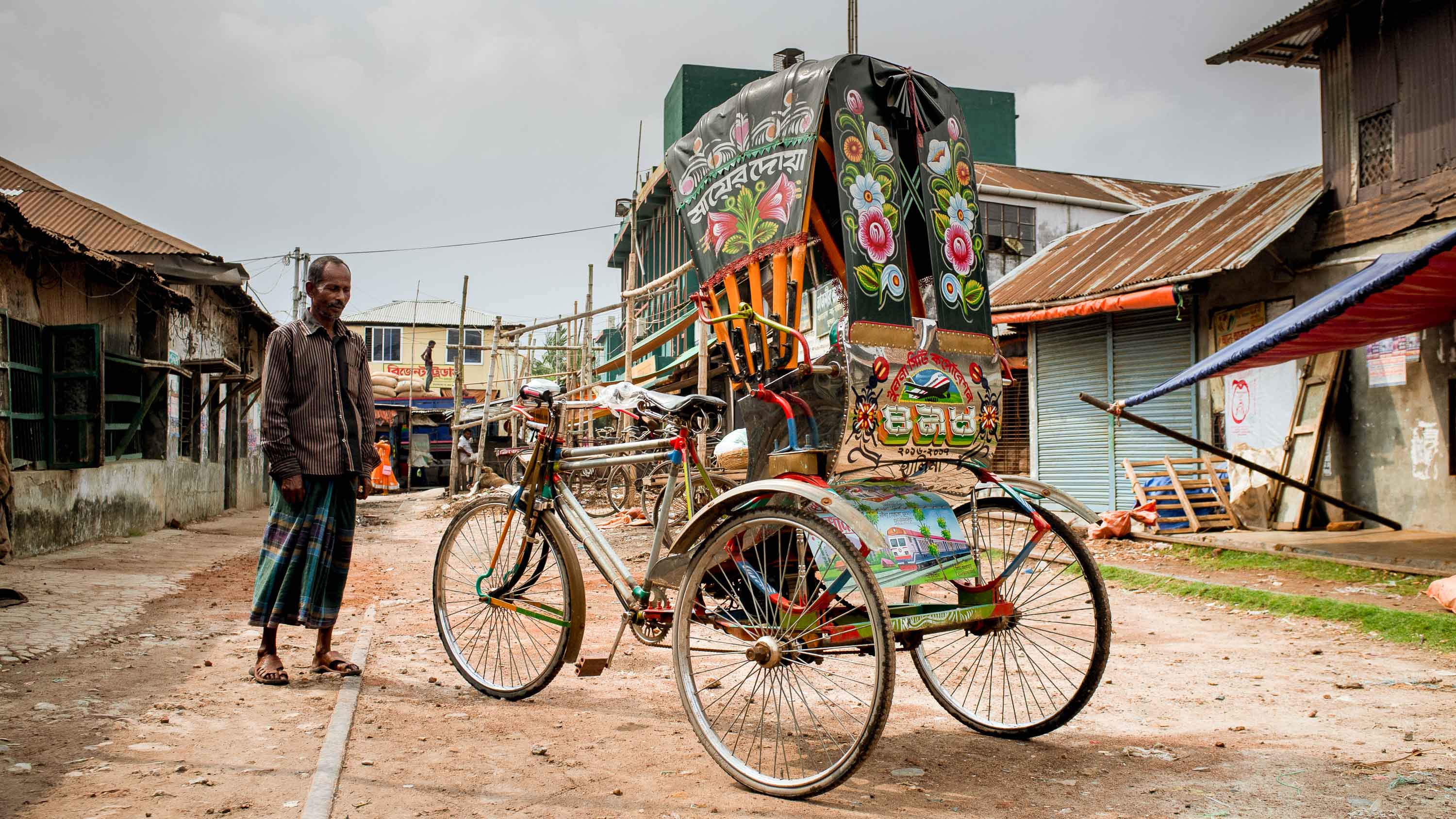In this detailed image set in what appears to be a small village in Eastern Asia, either India or Indonesia, a man stands on a dirt road amidst the rustic charm of an impoverished area. The buildings flanking the street are visibly aged and in disrepair, with rusting tin roofs and patchwork construction of metal fencing and concrete. A green building ahead shows signs of restoration, supported by handmade wooden scaffolding.

The man, adorned in a striped button-up shirt and a sarong-like garment with a green and purple pattern, stands next to a vividly decorated bicycle rickshaw, its canopy adorned with intricate paintings of flower blossoms in blue, pink, and green hues. The rickshaw presents a festive and ornate appearance, contrasting sharply with the surroundings.

In the background, life unfolds with diverse activities: a man is seen on a roof covered in sandbags, while a woman in a long yellow dress appears to dance. Further down, a business, possibly a restaurant, caters to the community. This evocative scene captures a blend of resilience and vibrancy amidst the evident poverty of the village.